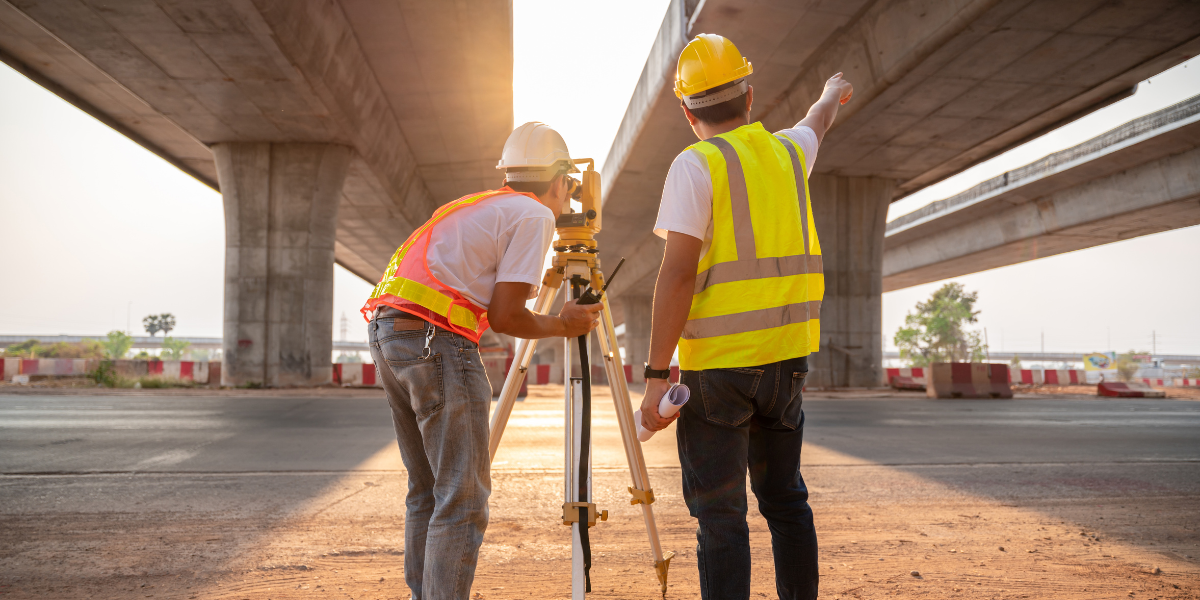The photo captures a bright, sunny day under multiple expansive bridge overpasses. In this scene, two construction workers, dressed in full safety gear, are immersed in their task. Standing between stout cement columns—white with splashes of red paint—the men seem focused on their surveying equipment, tripod-mounted and likely helping them with precise measurements. The worker on the right, dressed in a yellow helmet, white t-shirt, and a reflective yellow and gray vest, holds white papers in his left hand while his right hand points upwards. He also wears black pants and has a black device on his left wrist. The other worker, positioned to the left, sports a white helmet and a reflective orange and yellow vest. Both men's faces are turned away from the camera, emphasizing their concentration on the task at hand. The image highlights their methodical effort amid the structural grandeur of the bridge supports and overpasses looming above them.